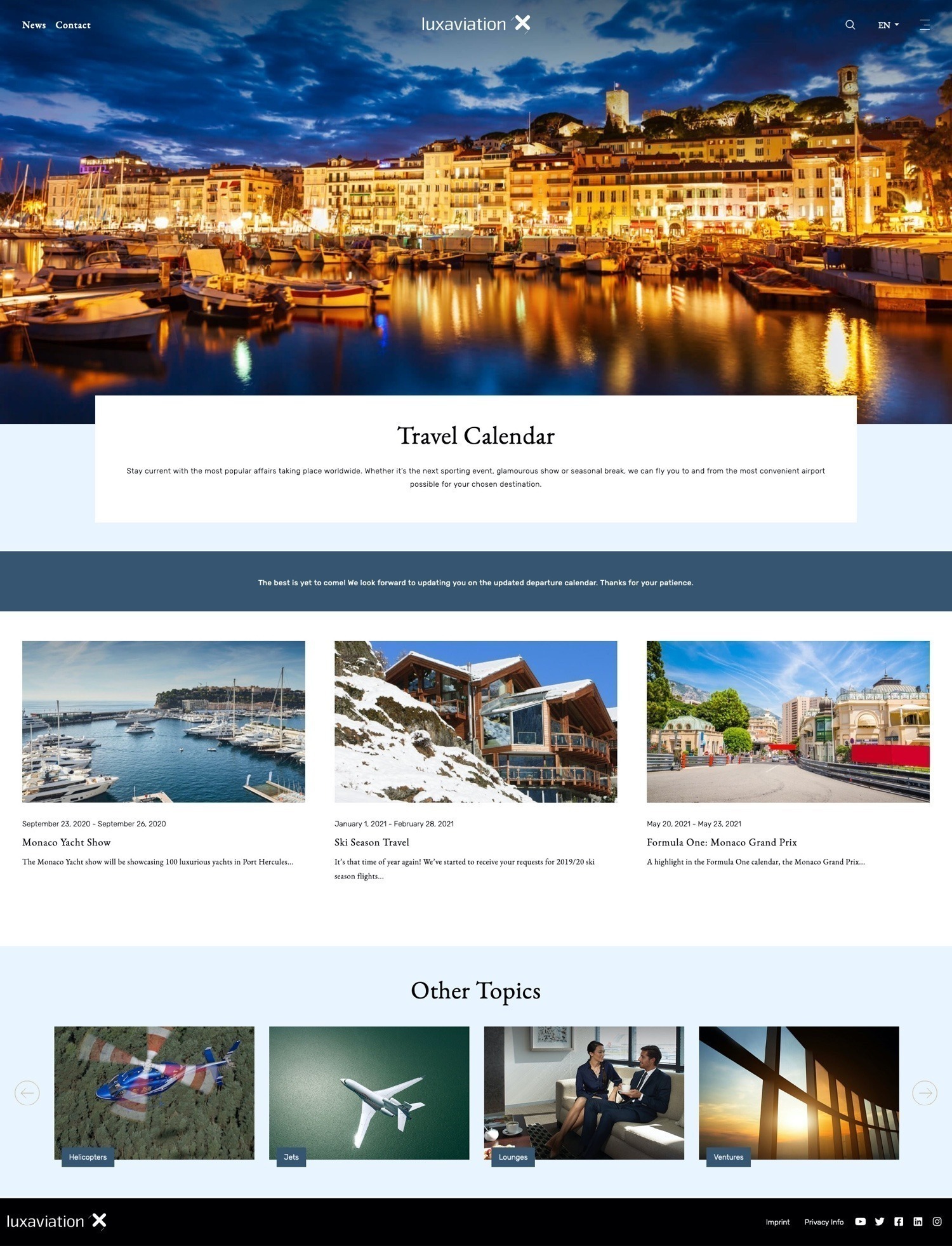The image prominently features the Luxaviation website interface, with a central screenshot highlighting the company's homepage. At the top left corner, navigational buttons labeled "News" and "Contact" are clearly visible. On the upper right, a search icon accompanies a dropdown menu displaying "EN" for language selection.

Beneath the central screenshot, a picturesque photograph showcases a panoramic view of a waterfront cityscape at dusk. The city's skyline, with its impressive array of buildings, forms a dramatic backdrop to a line of boats moored along the water.

Further down, a segment labeled "Travel Calendar" is presented, though the accompanying text is too small to decipher clearly. The lower portion of the image is divided into two rows of photographs, three in each row. The top row features, from left to right: additional boats on water, a cozy snow-covered cabin, and an image presumably related to a "Grand Prix" event, as indicated by the text.

The bottom row showcases an array of aviation-related images including helicopters, planes, a conference setting, and a scenic view captured from an airplane window.